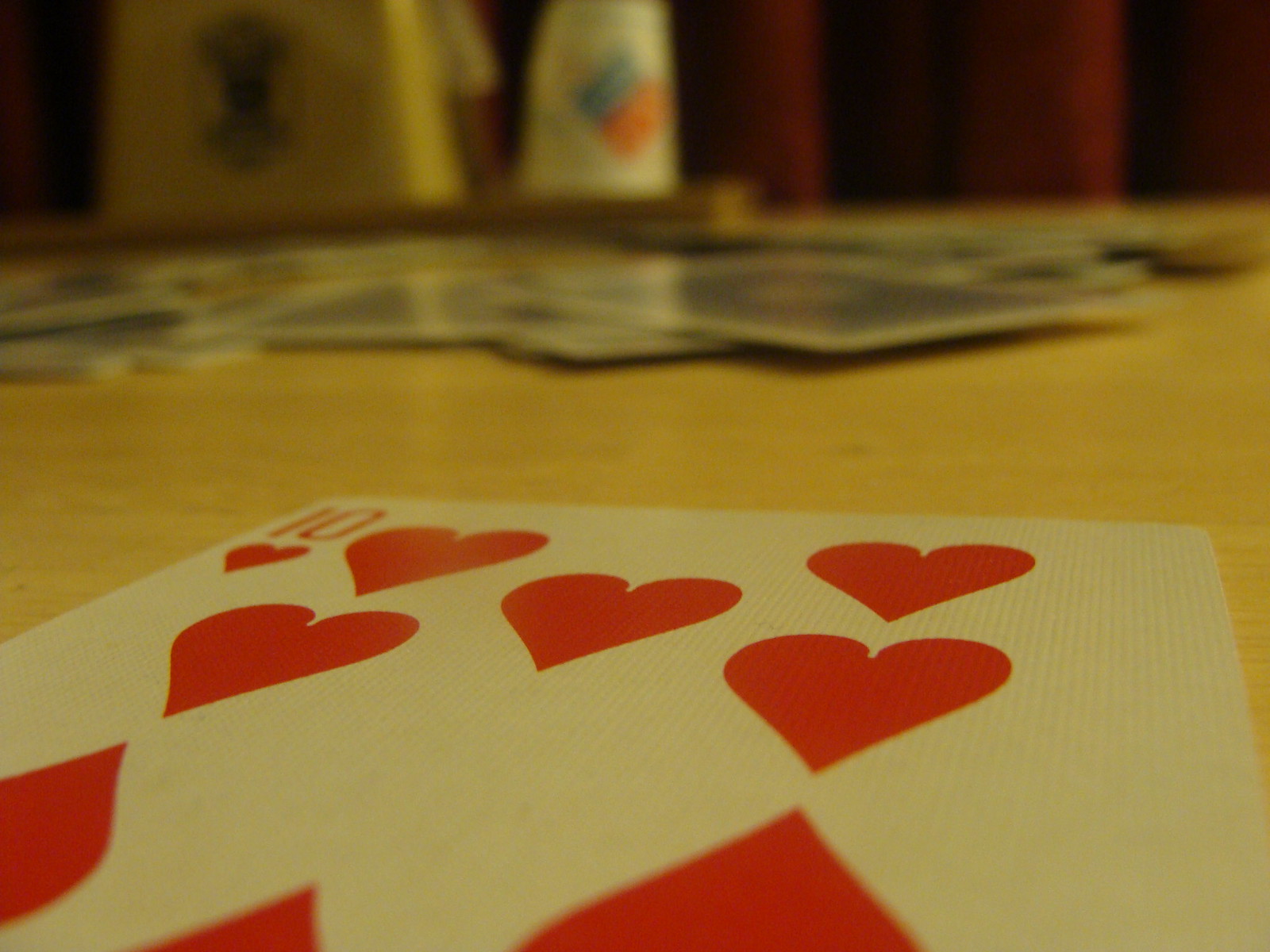In this photograph, a close-up shot focuses on a deck of playing cards scattered across what appears to be a kitchen table. The ten of hearts is prominently featured in sharp detail, standing out from the rest of the deck, which is blurred and dispersed across the scene. The background is out of focus, but faint colors suggest the presence of various objects, possibly including a red drape. Though difficult to discern clearly, there are hints of a blue canister and designs on other items in the background. The playing cards themselves have blue backs, adding a subtle contrast to the composition. The image captures a casual, possibly chaotic moment, centered around the ten of hearts.